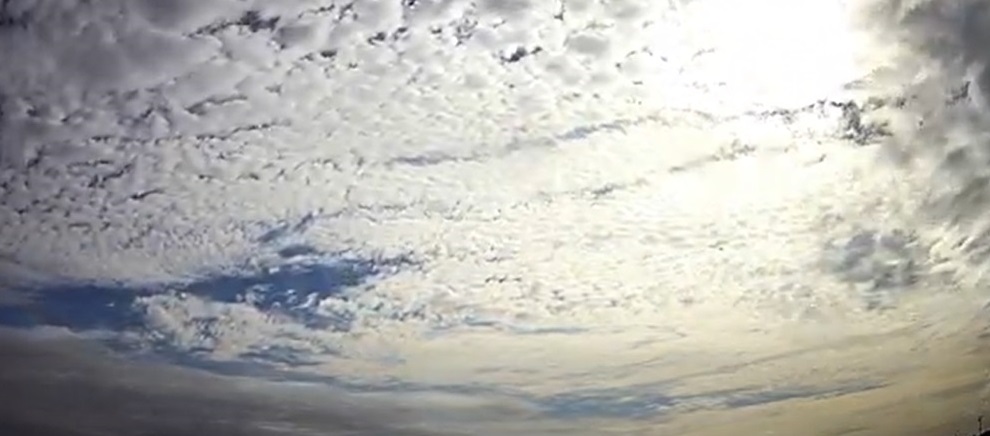This photograph captures a vast sky filled with a mix of thin, cirrus clouds and slightly thicker, darker gray clouds. Predominantly, the image portrays a single layer of these clouds stretching across the sky. The sun can be seen glowing behind the clouds in the top right corner, casting a white light through them, although the shape of the sun itself is obscured. The clouds are denser and grayer in this area, creating a contrast with the lighter, more scattered clouds toward the top left, where they break up to reveal patches of clear blue sky. Notably, in the bottom left corner, there are larger gaps between the clouds, allowing for broader views of the sky, which transitions from a darker blue at the top to a lighter blue at the bottom. The configuration of these blue patches alongside the clouds vaguely resembles the shape of eyeglasses. Overall, the clouds create a layered effect, swirling and thinning toward the bottom of the image, adding a dynamic texture to the scene.